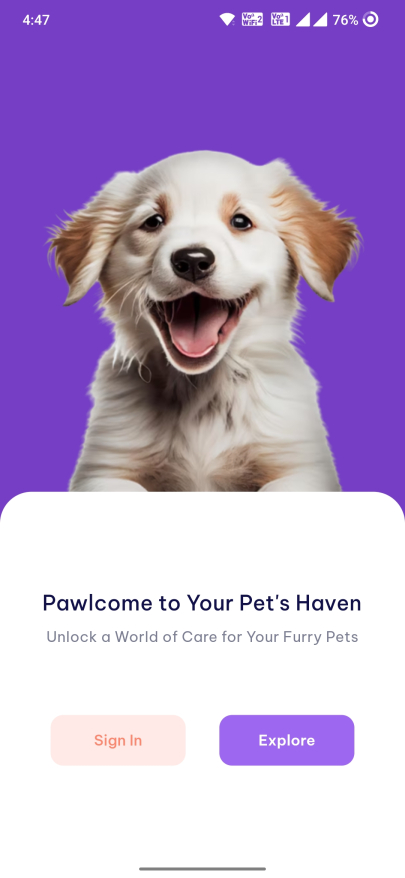This is a screenshot of a smartphone display. In the upper-left corner, the time reads 4:47, without specifying a.m. or p.m. Along the top edge of the screen, from left to right, there are icons for Wi-Fi signal, two cell phone signal strength indicators, and a battery level showing 76% in the upper-right corner.

The main portion of the screen features a vibrant purple background. Dominating the screen is a cheerful, white puppy with brown ears, brown spots around its eyes, and a brown patch on its chest. The puppy appears to be smiling, likely due to computer-generated imagery, and has a shiny spot on its black nose.

Below the puppy, against a white field, the text reads, "P-A-W-L-C-O-M, welcome to your pet's haven. Unlock a world of care for your furry pets." Beneath this text are two distinct buttons: a pink sign-in button with orange letters on the left, and a purple explore button with white letters on the right. A gray bar spans the very bottom of the screen.